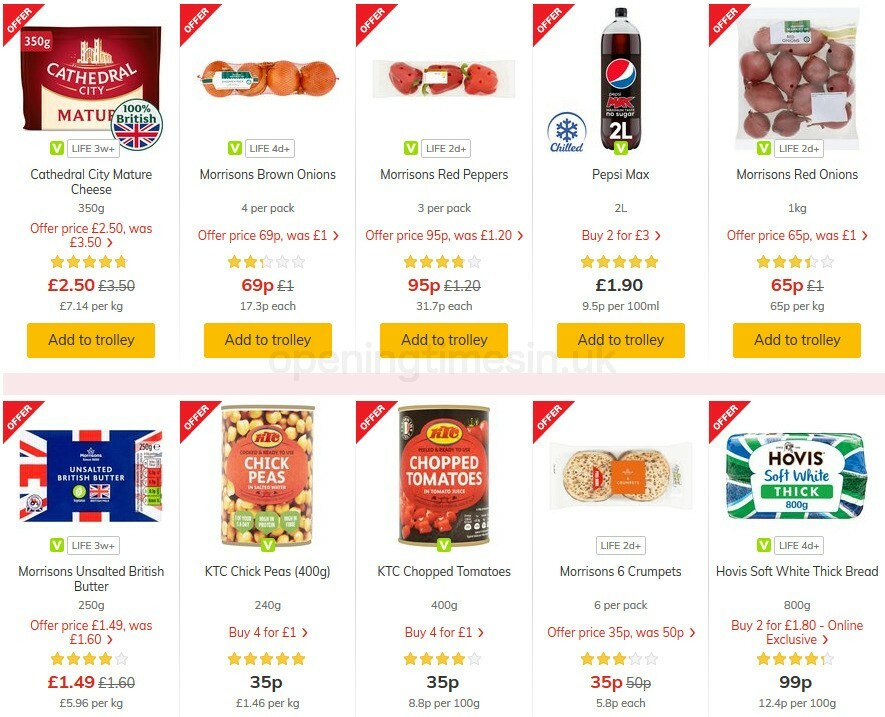This image is a detailed view of a food e-commerce website showcasing various food items on sale. Each product has a prominent red banner in the upper left corner indicating it's part of a special offer. 

Starting with Cathedral City Cheese, originally priced at $3.50, it is now offered for $2.50. Next are onions priced at $0.69, followed by a special offer for Morrison's Red Peppers at $0.95.

Additional items include a 2-liter bottle of Pepsi, red onions, unsalted British butter, KTC Chickpeas, KTC Chopped Tomatoes, and Morrison’s Crumpets. Another item highlighted is soft, white, thick bread. This bread is particularly noted as an online exclusive with a special deal - buy two for $1.80.

The KTC Chickpeas and KTC Chopped Tomatoes are on a buy four for a dollar special, and the Morrison’s Crumpets are priced at $0.35 each in the offer. Lastly, an item listed at the bottom is priced at $1.49, down from $1.69. 

The prices appear to be using a foreign currency, suggesting this website could be based outside the United States. The detailed promotional pricing and the variety of items suggest a comprehensive sale event aimed at offering value on everyday groceries.